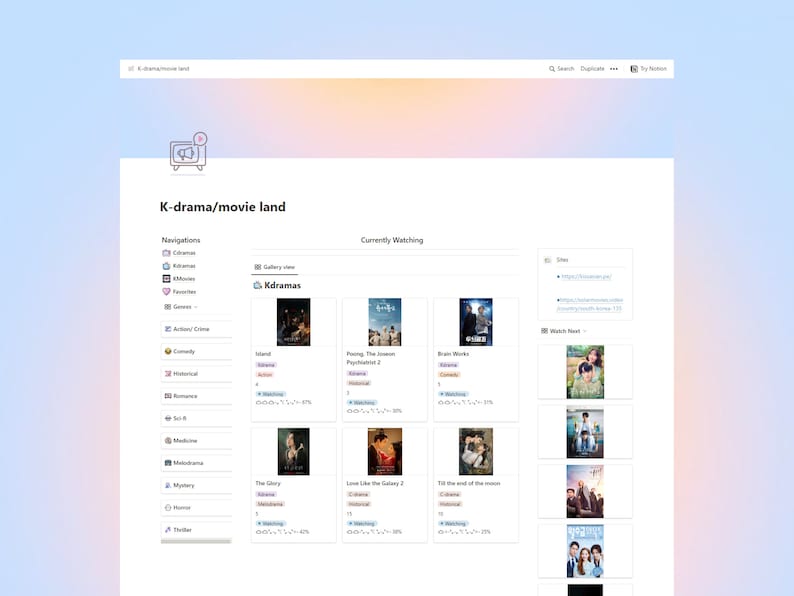The image appears to be a screenshot of an application interface on a computer screen, designed for K-Drama enthusiasts. The background features a soothing aurora-like blend of blue and orange-pink hues, evocative of the Northern Lights. At the top of the screen is a prominent white text box with the title "K-Drama Movies Land" written in elegant black ink. To the right of this text box are several function buttons, including "Options," "Search," and "Duplicate." 

Below the main header, the interface has a large white section overlaying the aurora backdrop, which also reads "K-Drama / Movies Land" in the same black ink. This area includes a navigation menu with difficult-to-read text due to its small size, listing categories such as "Favorites" and others. The app interface further features a "Currently Watching" section, displaying the user's ongoing viewing activities, likely personalized for easy access to continue watching their favorite K-Drama content.